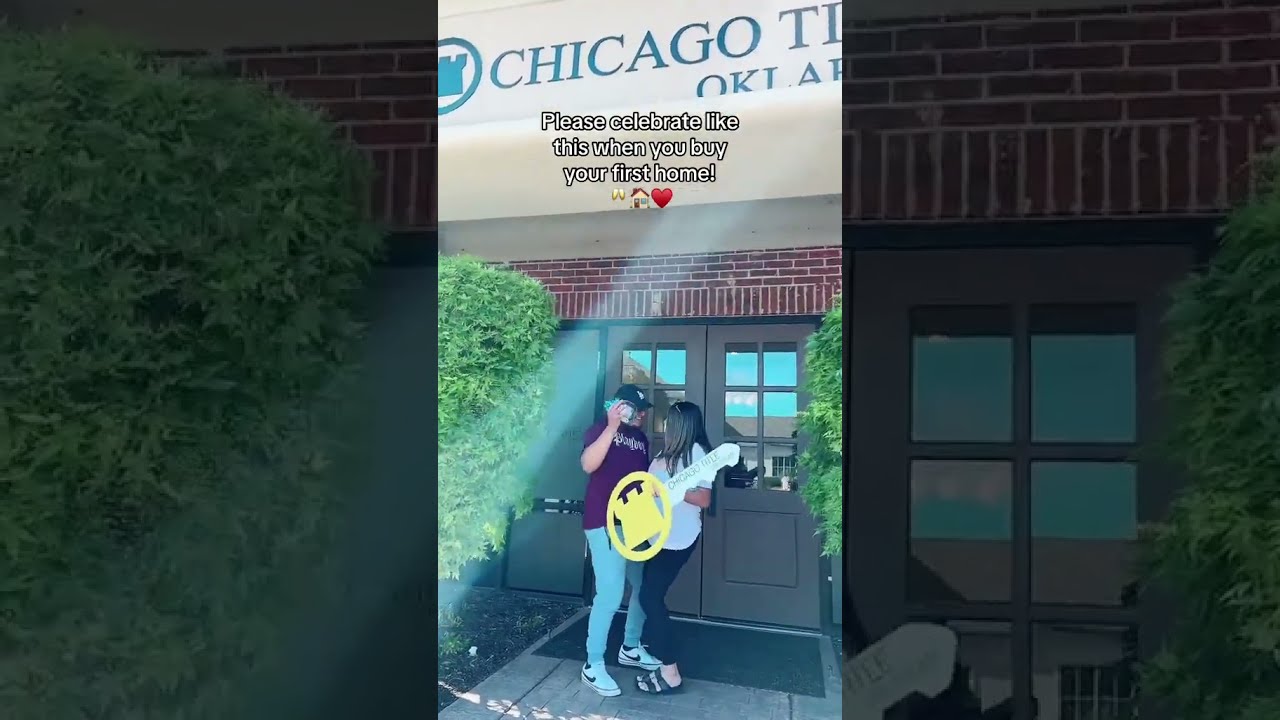The image is a vertical collage of three photos, each layered to provide a comprehensive and cohesive visual story. The central section showcases a joyful moment between a man and a woman, both standing in front of a brick building with two grey doors featuring six square windows each. On either side of these doors are leafy trees and bushes adding a touch of greenery to the scene. The man, dressed in a ball cap, maroon shirt, light-colored jeans, and tennis shoes, is looking happily towards the woman. She is attired in a white shirt, dark pants, and sandals, holding a large, cutout key in a celebratory pose. Their bodies are slightly curved towards each other as if frozen in a dance.

Above the pair, in the middle part of the photo, are playful texts and emojis that read, "Please celebrate like this when you buy your first home," accompanied by icons of wine glasses, a home, and a red heart. On the upper frame, partially visible text spells out "Chicago" and fragments of additional words. The original images, used to create this collage, have dark, almost film-like filters with the first and last visuals emphasizing the brick wall and grey doors, adding cohesion to the collage's aesthetic. A welcome mat lies at their feet, grounding the scene in a warm, inviting tone.